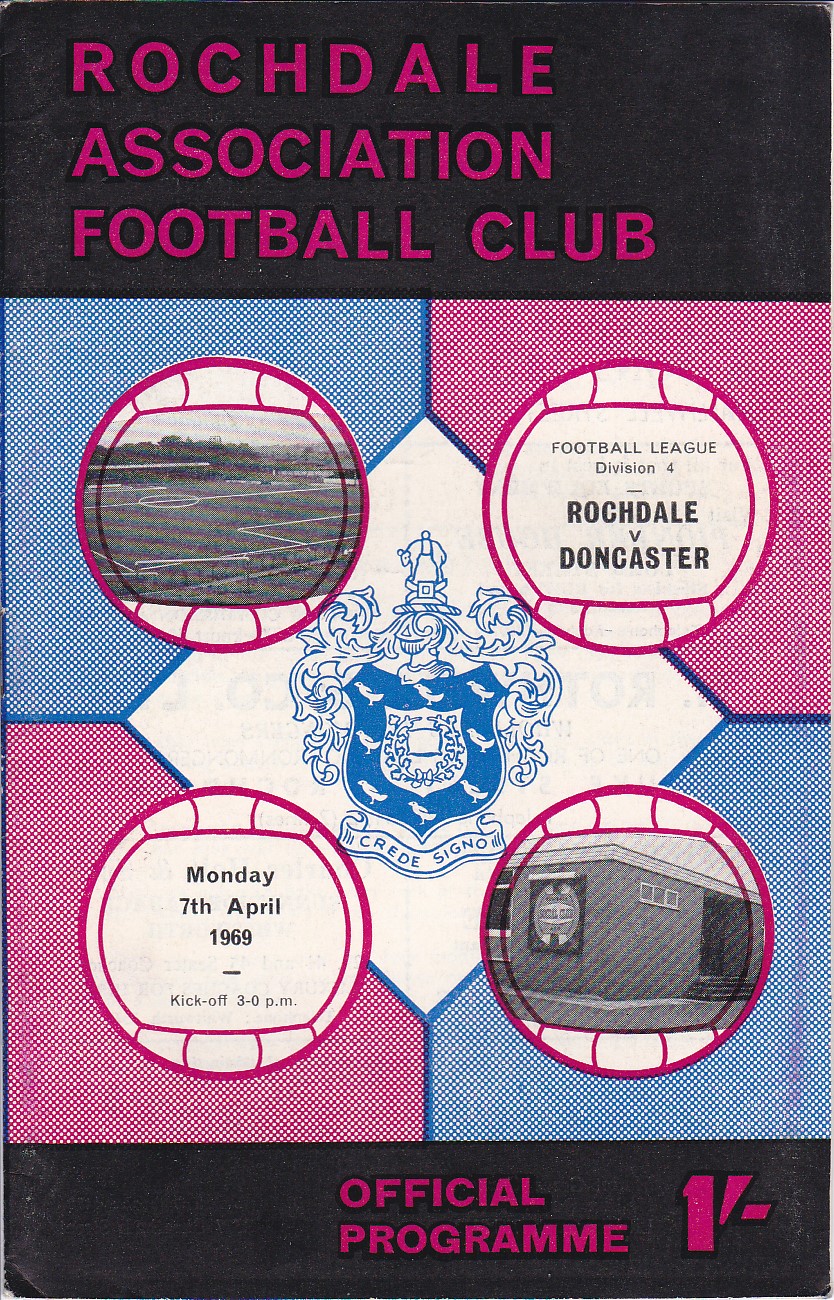This color image serves as the cover of a sports program, distinguished by its vibrant pink, blue, black, and white hues. Dominating the top section is a black bar showcasing pink text that reads "Rochdale R-O-C-H-D-A-L-E Association Football Club." At the bottom, another black bar features the text "Official Program" and the number "1." Central to the design is a blue crest set against a white background, surrounded by four interconnected circles in pink, each resembling a soccer ball outline.

The top left circle contains a black and white photograph of a soccer field, while the top right circle displays the text "Football League Division IV, Rochdale vs. Doncaster." The bottom left circle indicates the match date and time: "Monday, 7th April, 1969, kickoff at 3 p.m." The bottom right circle features an image of a one-story building, although details on the building are minimal. Overall, the cover blends vibrant colors and clear sections, creating an eye-catching preview to the matches.